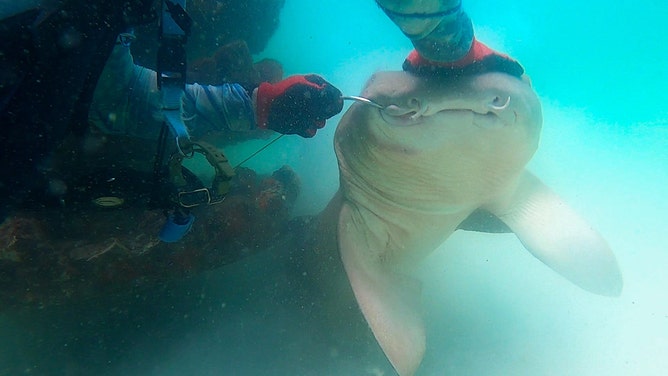In an underwater photograph, a man with red and black gloves grips a hook that pierces the front nose of a shark, his other hand resting on the top of the shark’s head. His face remains obscured as he manipulates the steel device, possibly attempting to free the shark from the hook. The scene reveals the shark’s grey and white underbelly, with visible fins and mouth. The water around them is blurry and filled with debris, indicating a disturbed environment. Behind the man, some underwater vegetation is visible. A tool belt laden with equipment is seen to the left, suggesting the man is equipped to handle this underwater task, likely aimed at rescuing the shark from its plight.